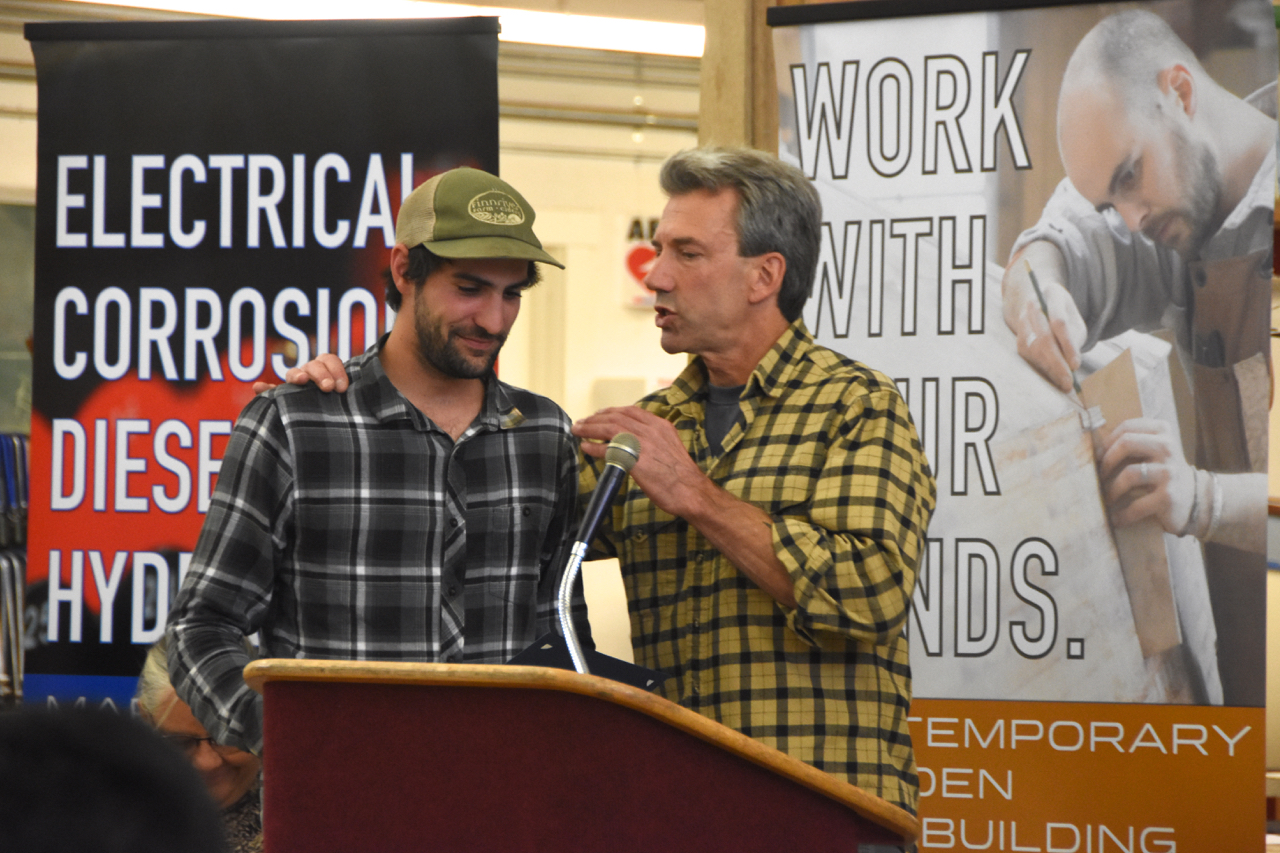The image captures a scene from what appears to be a presentation or conference. Two men are standing at a wooden podium equipped with a silver stand and a black microphone. The man on the right, who is slightly older with black and gray hair, is wearing a dark yellow and black plaid button-up shirt over a gray t-shirt, with his sleeves rolled up. His right hand rests on the left shoulder of the man next to him, and his left hand is raised as if he is explaining something. The man on the left, younger with dark facial hair, is donning a green and white trucker's hat and a black, gray, and white plaid button-up shirt. He stands at the left-hand side of the podium, slightly smirking and looking down. In the background, a couple of posters can be seen, one discussing electrical corrosion and diesel, and another promoting trades like carpentry with phrases about working with your hands. An older woman is seated behind them to the left. The overall setting emphasizes a focus on practical trade skills and hands-on professions.